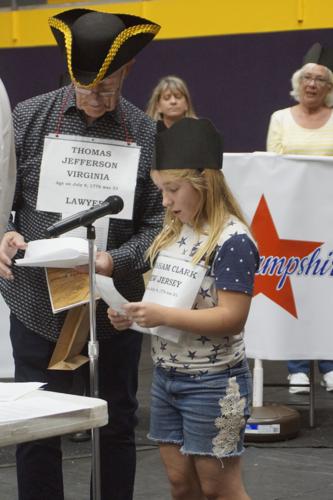This photograph captures a stylized Revolutionary War-era reenactment likely taking place in a school setting. Central to the scene, an older man dressed as Thomas Jefferson, wearing a tri-point hat and a black shirt, stands at a microphone. A banner around his neck reads, "Thomas Jefferson, Virginia, Lawyer." Beside him, a young girl, approximately 9-10 years old, dons a black paper hat with a wavy top. Her shoulder-length blonde hair complements her patriotic outfit of a short-sleeved shirt, white with blue stars on the center and blue sleeves adorned with white polka dots, paired with denim shorts. She wears a sign around her neck indicating her character is someone named Clark from New Jersey. Both of them hold papers, seemingly reading from them.

In the background, two women also in costume watch the proceedings; one older woman wearing a paper hat similar to the girl's stands partially obscured behind a banner with "Hampshire" visible, while a younger woman stands further back. The background banner, adorned with a red star and the partially visible word "championship," suggests a celebratory or competitive framing to the reenactment event.